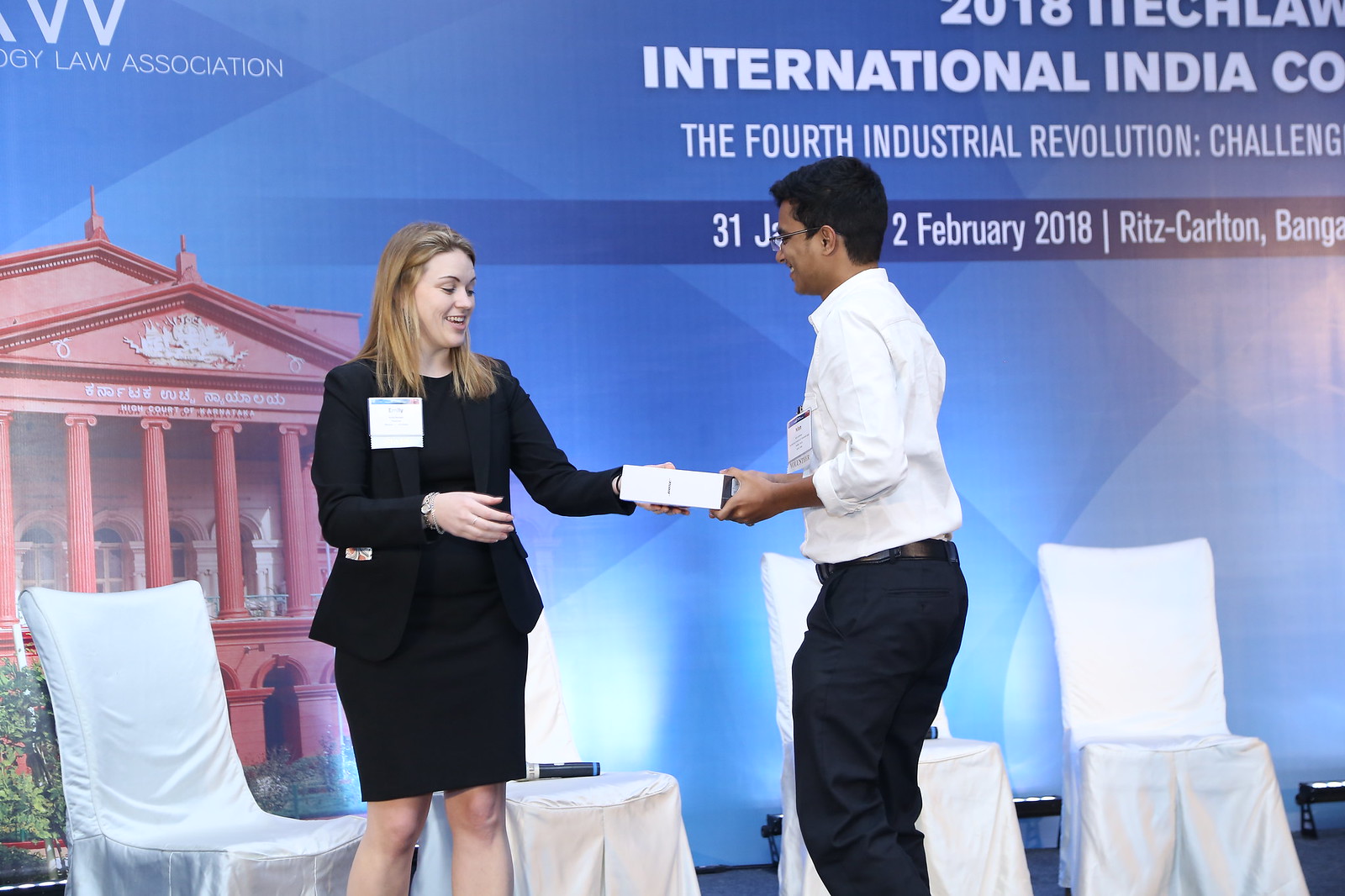The image features a stage setting where a woman on the left and a young Indian man on the right are engaged in a ceremonial exchange. The woman, who appears to be in her 30s, is Caucasian with medium-length light brown hair, and she is dressed in a professional black suit. She stands facing slightly to her right, extending her left hand to receive a box from the man. The man has very short black hair and is dressed in a white long-sleeve dress shirt with dark (possibly black or navy blue) pants. He hands over the box with both hands and wears glasses. Both of them are wearing large name tags pinned to the left side of their shirts, almost the size of a CD case. 

In the backdrop, there is a display that includes text mentioning "International India Conference," "The Fourth Industrial Revolution," and specific dates "31st January to 2nd February 2018." It appears to be an advertisement banner for the event at the Ritz Carlton. Additionally, there are white chairs and tables covered with white slipcovers on the stage behind them. The backdrop also features a red building with columns on the left and a blue background on the right, with the words “Law Association” partially visible in the upper left corner. Both individuals are smiling, adding a sense of formality yet amicable interaction to the scene.